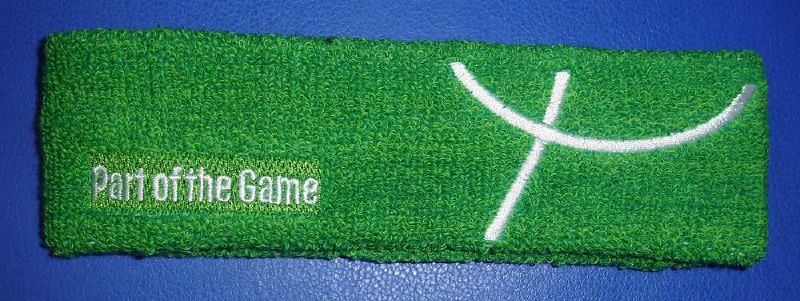This indoor photographic advertisement features a green wristband or headband that resembles a block of astroturf placed on a texturally rich blue background. The rectangular headband has a terrycloth-like texture and is detailed with two intersecting white embroidered lines—one vertical and the other horizontal—that cross in the middle, creating an almost cruciform shape. The curved top and diagonally angled bottom of the white crossing lines add a unique visual element. Positioned to the left of the wristband is the phrase "part of the game," also embroidered in white.